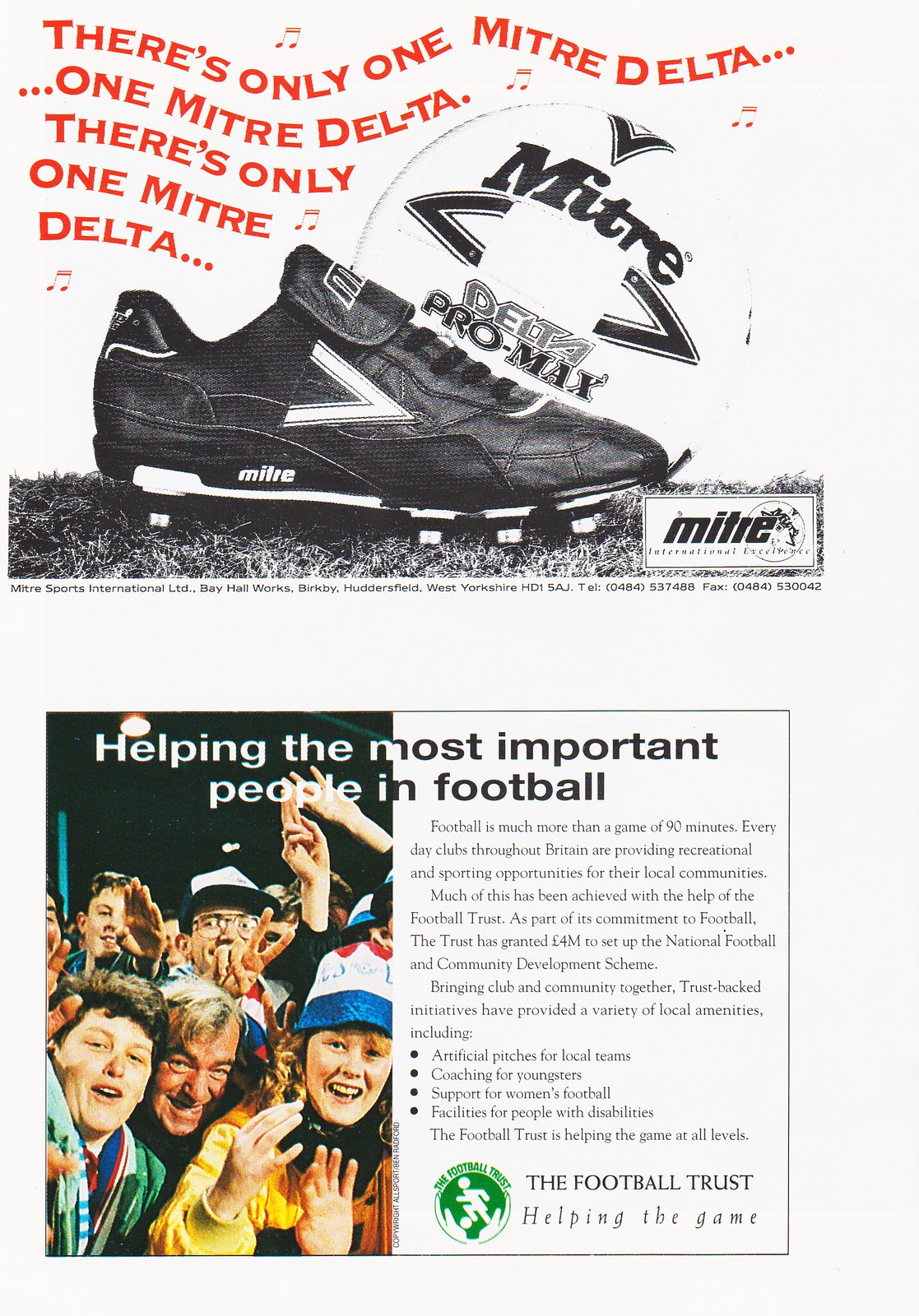This scan appears to be from a sports magazine or program and features two stacked advertisements. The top advertisement is predominantly black and white, with a distinct red text reading, "There's only one Mitri Delta. One Mitri Delta. There's only one Mitri Delta." The text is formatted in a wavy, musical style with accompanying music notes. Below this text is a black-and-white image depicting a soccer cleat on turf with a soccer ball branded 'Mitri' behind it.

The bottom advertisement is in color, highlighting a group of fans at a soccer game. The left side of the ad features a photograph of a man surrounded by children, mostly showing their eager faces. The right side switches to a white background with the text, "Football is much more than a game of 90 minutes. Every day clubs throughout Britain are providing recreational and sporting opportunities for their local communities." This text transitions from white to black lettering and emphasizes community support in football. Beneath it is the slogan, "The Football Trust - helping the game," along with the Football Trust's green logo.